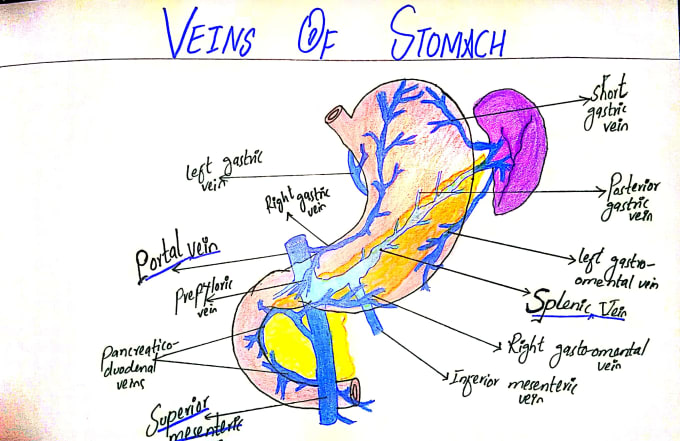This is a detailed, hand-drawn anatomical diagram of the veins of the stomach, created using pencil and colored pencils. The image features a side view of the stomach, outlined with fine-lines and shaded in pink, with veins depicted in blue. The veins prominently branch out across the stomach, with six large veins extending in a branching fashion across its exterior. An oval-shaped purple organ, likely the spleen, is connected to the right side of the stomach by these veins. The veins are meticulously labeled in black handwritten text, identifying each one, including the left gastro vein, right gastro vein, portal vein, preptoric vein, pancreaticoduodenal veins, superior mesenteric vein, anterior mesenteric vein, right gastro-omental vein, splenic vein, left gastro-omental vein, posterior gastric vein, and short gastric vein. Lines extend from the labeled veins to specific parts of the diagram for clarity. The drawing is set against a slightly off-white background, and at the top, in large blue handwritten text, it reads "Veins of Stomach." The detailed and colorful presentation suggests it may have been created as a study aid for someone learning about stomach anatomy.